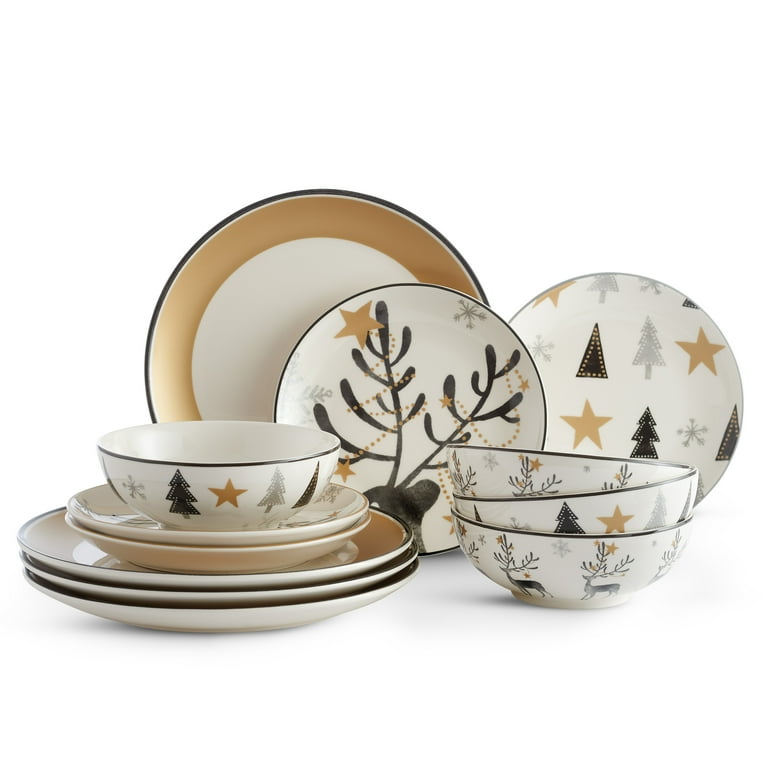This picture features a holiday-themed dishware set meticulously arranged for a product image against a pure white backdrop. The set includes four bowls, four smaller plates, and four larger plates, all sharing a unified festive design likely intended for Christmas or winter celebrations.

At the center of this arrangement is the main larger plate, prominently showcasing a reindeer with its antlers adorned with gold stars and what appear to be ornament-like dots, contributing to an aesthetic resembling holiday ornaments or decorations. Surrounding this central plate are additional plates featuring designs of Christmas trees in dark green and white, gold stars, and silver snowflakes, enhancing the festive theme.

To the left, three bowls are stacked, while a fourth sits separately. Positioned upright and neatly behind these, ensuring full visibility, are three additional bowls, echoing the same holiday patterns of reindeer, trees, stars, and snowflakes.

The color scheme throughout the dishware incorporates dark green borders, white interiors, and accents of pale gold, maintaining a harmonious yet festive appearance that would grace any holiday table setting. The entire setup is thoughtfully staged, highlighting the cohesive design and intricate detailing of each piece in the set.